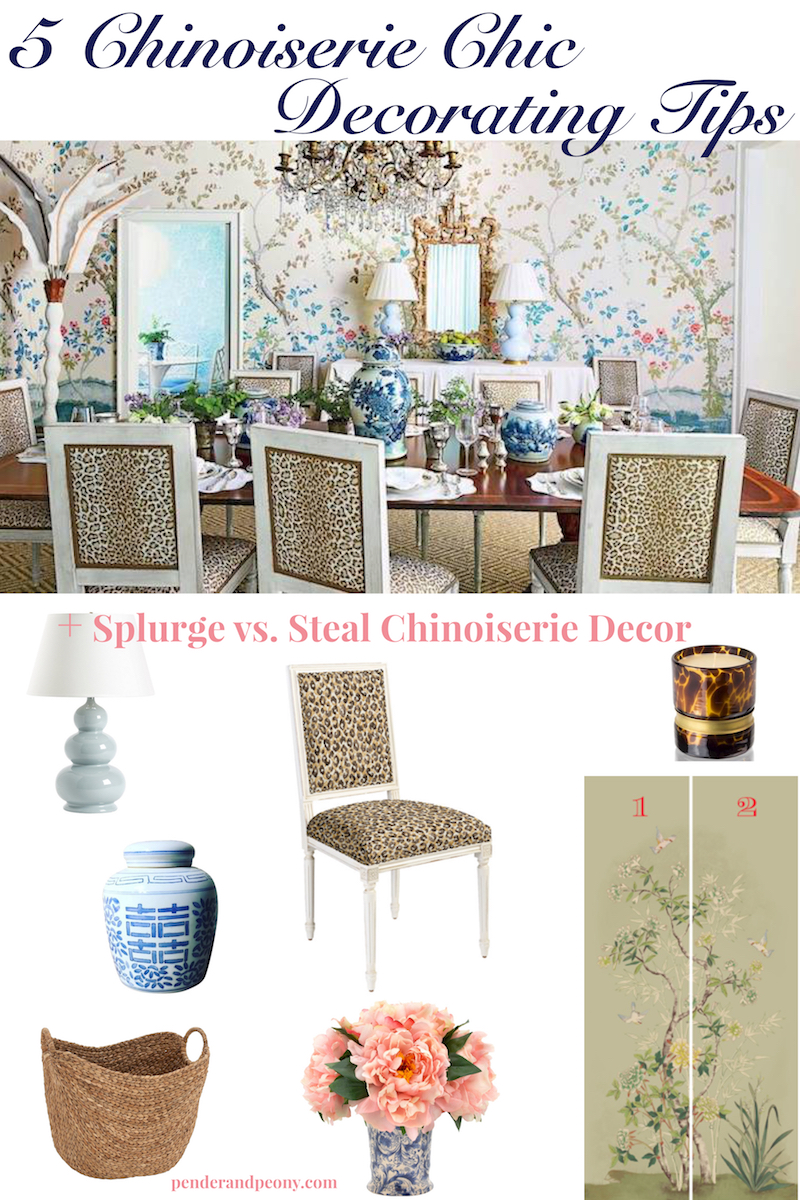The image from penderandpeony.com, titled "Five Chinoiserie Chic Decorating Tips," showcases an elegant dining room adorned with chinoiserie elements aimed at achieving luxurious decor without overspending. The graphic features a cursive title and presents a dining area with a mahogany table surrounded by at least six cheetah print chairs. On the table are various vases with blue prints on a white base, along with plants, contributing to the chic aesthetic. There's a dresser against the wall holding two lamps and a mirror, with floral and tree-patterned wallpaper enhancing the setting. Below this main image, there's a "splurge versus steal" section that contrasts high-end chinoiserie decor items with their more affordable counterparts, including a lamp, additional vases, a wicker basket, and a room divider. The website link, penderandpeony.com, is prominently displayed at the bottom, guiding viewers to explore further how they can infuse their homes with chic chinoiserie style while remaining budget-conscious.